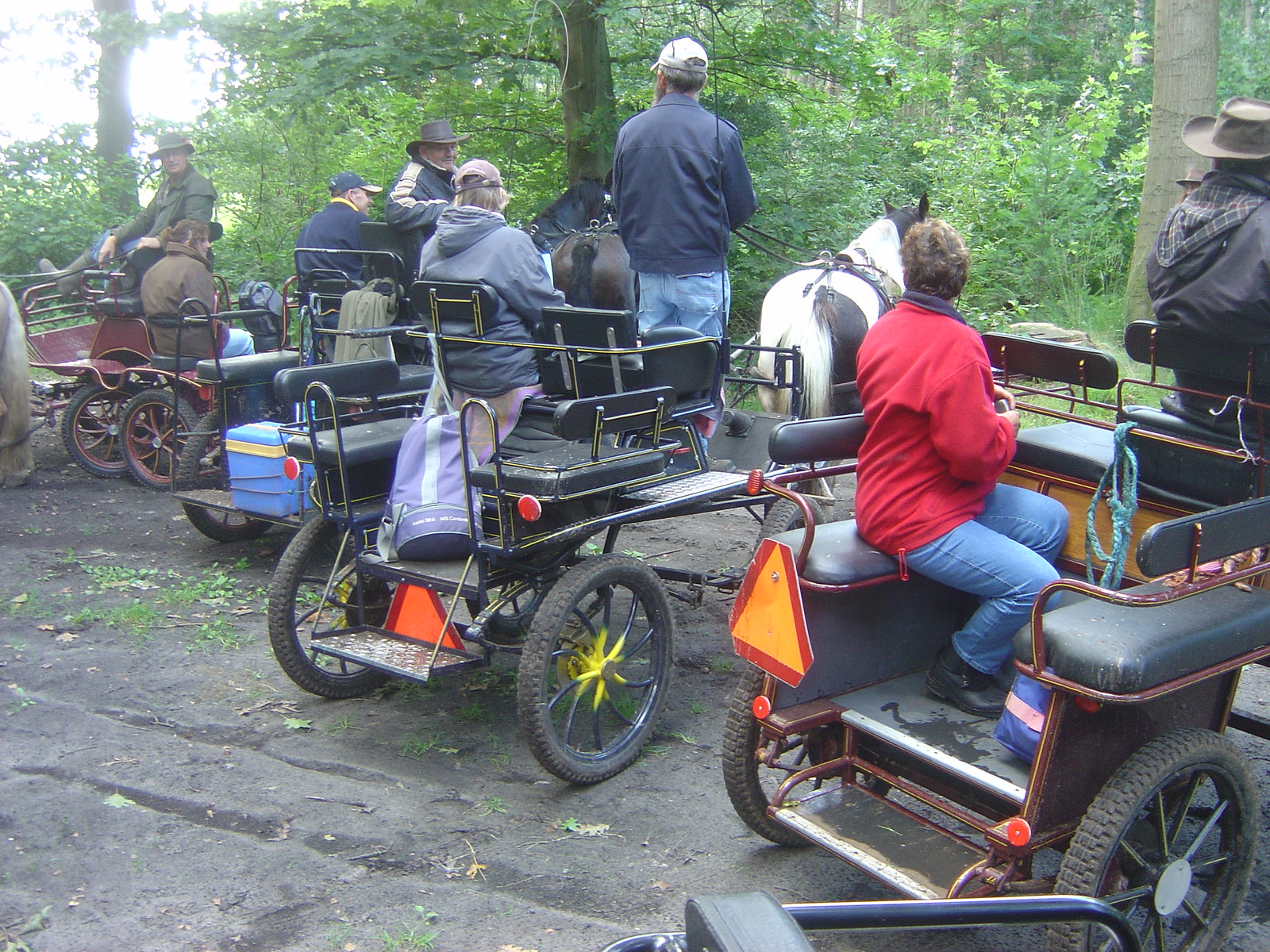The photograph captures a lively scene in a northern American forest, where the dirt and leaf-covered ground sets a natural backdrop for several horse-drawn buggies. The image features four carriages, each pulled by a single horse and constructed with metal frames, wooden seat backs, and rubber tires. These modern-looking buggies have seats that sometimes face sideways, and each sports a yellow and red warning triangle on the back. The buggies carry a range of passengers, with some occupied only by the driver and others hosting additional riders, alongside coolers and luggage.

On the far left, a light gray tail of a horse pulling a red cart is visible. In the background, a black horse pulls a dark cart, while a bay horse is hitched to another dark carriage nearby. To the right, a reddish-black cart with two passengers—one driver and one rider—is seen, although the horse is not visible. The center cart, driven by a person who stands while conversing with others, is pulled by a sturdy, paint horse, possibly an Irish cob.

Amidst the greenery and patches of the light-colored sky peeking through the trees, the attire of the passengers stands out. Many wear denim and dark blue or gray jackets, with some donning brown and white hats. A woman in a red jacket and blue denim pants adds a splash of color to the scene. The setting is enhanced by the intricate details on the carriages, from their yellow spoke-painted tires to the various items hanging at the back, showcasing a harmonious blend of natural beauty and human activity.